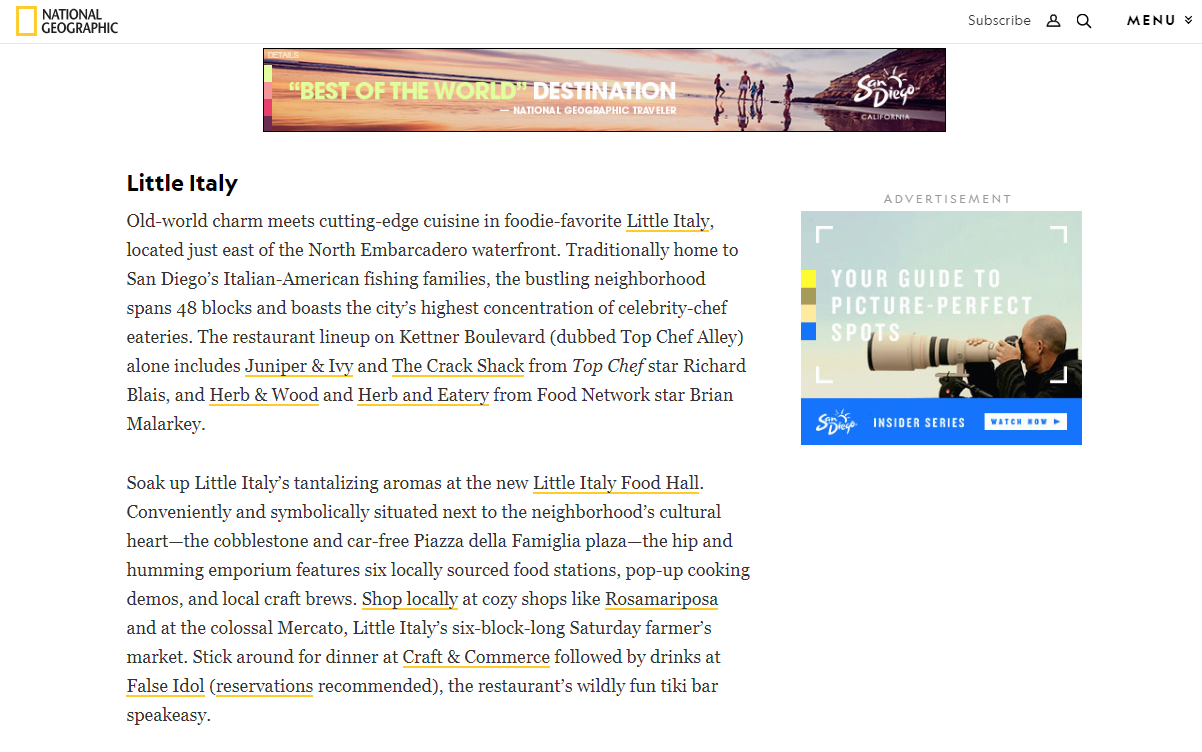This image is a screenshot from the National Geographic website, identifiable by the "National Geographic" logo in the top left corner, accompanied by a distinctive hollow yellow square. The top right corner features options such as "Subscribe," a person icon, a magnifying glass icon, and a "Menu" drop-down arrow.

The webpage contains two advertisements. The top ad is a long rectangle promoting "The Best of the World Destinations," depicting people on a beach during sunset. The second ad is located to the right and showcases a person gazing through a telescope with the tagline, "Your Guide to Picture-Perfect Sports – Insider Details."

The main content is an article headlined in bold as "Little Italy." The article's body text describes the neighborhood as a blend of old-world charm and modern culinary innovation, making it a favorite among food enthusiasts. Little Italy, positioned just east of the North Embarcadero waterfront, has historically been home to San Diego's Italian-American fishing families. The vibrant 48-block area boasts the city's highest density of celebrity chef-run restaurants. A notable culinary hotspot is Kettner Boulevard, which features eateries such as Juniper & Ivy and The Crab Shack. The article highlights the dynamic, bustling nature of the neighborhood.